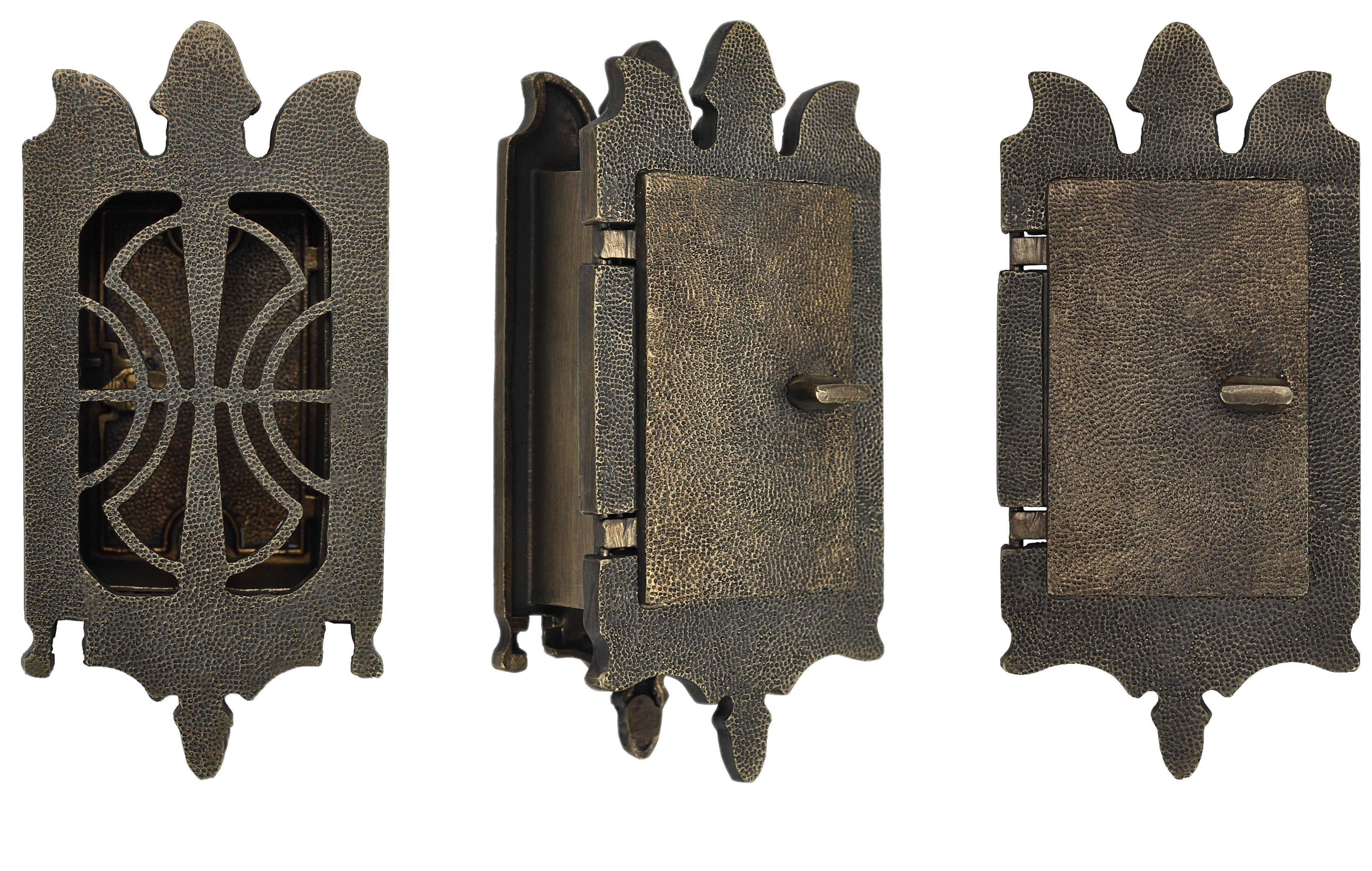The image presents three different views of an intricately designed metal structure, displaying various stages of a door being closed or opened. The structure exhibits a weathered, bronze patina, enhancing its vintage aesthetic.

On the left side, the first view reveals the structure with visible openings and ornate designs, allowing a glimpse into its slightly darker interior. The middle view offers a perspective on a different side, showcasing its three-dimensionality, with sculpted elements that provide an appearance of waves or curves. This view also highlights a door, featuring hinges and a slightly brighter bronze finish that contrasts elegantly with the rest of the piece.

Finally, the right-hand view provides a direct, front-facing perspective of the door, complete with visible hinges and a small latch or handle, all rendered in the same elegant bronze. The design elements suggest influences of gothic architecture, giving the entire piece an air of antique craftsmanship. The structure may function as a decorative box or cabinet, possibly for items like jewelry, enhancing its functional and aesthetic appeal.